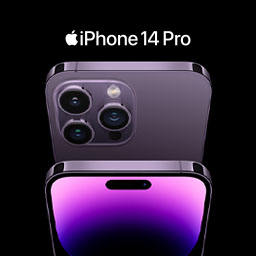This image is a promotional screenshot from Apple, showcasing the iPhone 14 Pro. It appears to be from one of Apple's annual events where they reveal new devices. The background is black, highlighting the advertisement's sleek design. At the top center, there's a white Apple logo with a distinctive bite mark on the right side. To the right of the logo, the text "iPhone 14 Pro" is prominently displayed. Below the text, there are images of the iPhone 14 Pro, both front and back, in a striking purple color. The back of the phone features three camera lenses and a flash module, while the front displays the screen with a pill-shaped cutout for the camera at the top. The overall design emphasizes the sophisticated aesthetics and advanced features of the iPhone 14 Pro.